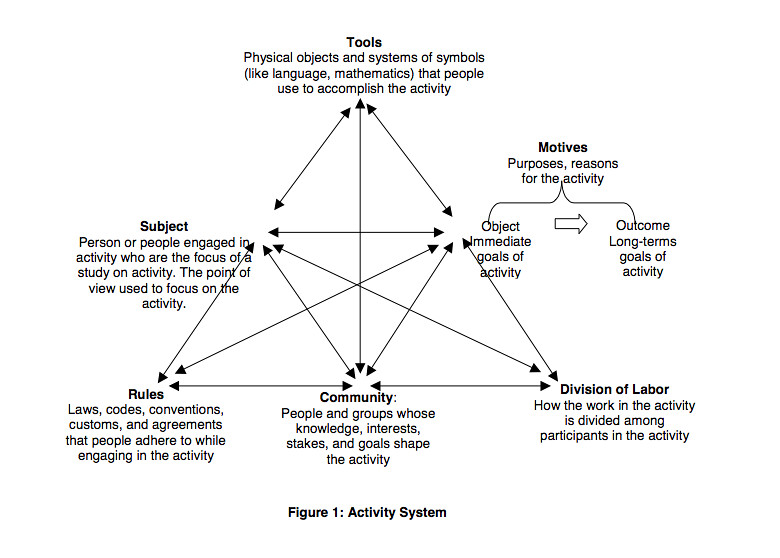The image is a detailed diagram labeled "Figure 1: Activity System," set against a white background with black text. At the center of the diagram is a large triangle interconnected by a network of arrows, indicating the relationships between different components. 

- **Top of the Triangle (Tools):** At the apex is labeled "Tools," which are defined as physical objects and systems of symbols, such as language and mathematics, that people use to accomplish activities.
- **Bottom Left Corner (Rules):** This corner highlights "Rules," the laws, codes, conventions, customs, and agreements people adhere to while engaged in activities.
- **Bottom Right Corner (Division of Labor):** Here, it reads "Division of Labor," detailing how work and activities are divided among participants.

Each corner and side of the triangle contains a descriptive paragraph. 

- **Left of the Triangle (Subjects):** This section is titled "Subjects" and describes persons or people engaged in activities who focus on a study or activity.
- **Right of the Triangle (Motives):** Labeled "Motives," this part explains the purposes or reasons for the activity. It includes a bracket dividing "Object" (immediate goals) and "Outcomes" (long-term goals).
- **Center of the Triangle (Community):** In the middle, "Community" is defined as people and groups whose knowledge, interests, stakes, and goals shape the activity.

The interconnected arrows emphasize that these elements are interrelated, forming a cohesive system.